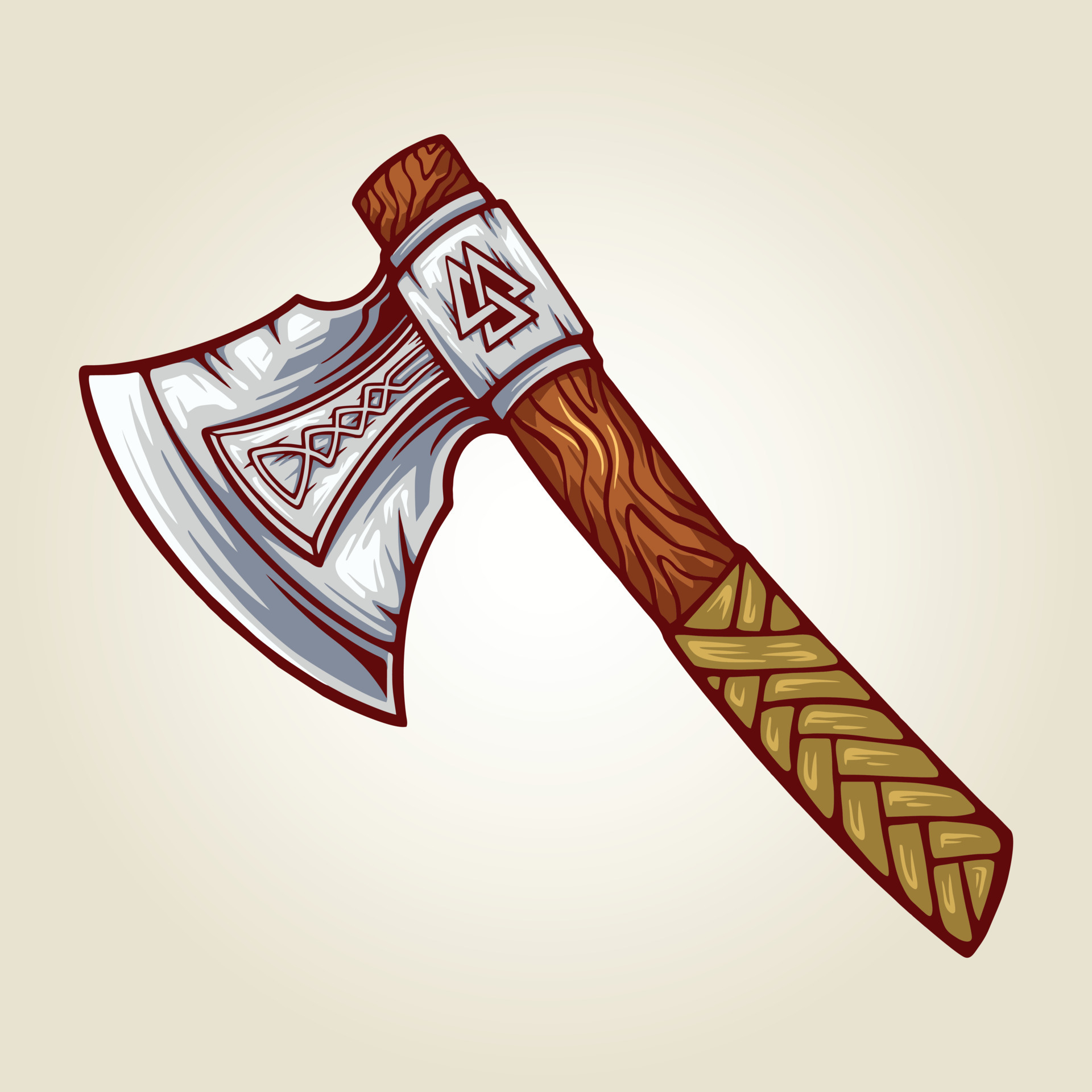This is a square-shaped image featuring a digitally-created drawing of what appears to be a Viking axe, possibly designed for a video game. The handle starts at the lower right portion of the image and rises towards the upper left, with the blade's edge pointing downwards to the lower left corner. The handle is wooden, with its lower half wrapped in a cloth or leather material that has a light brownish-green hue. The upper half of the handle is plain wood, characterized by a dark brown color.

The metallic blade of the axe is light gray with silvery highlights and features intricate engravings, including a notable Celtic triple triangle design and other geometric shapes resembling spiral triangles. These engravings run along the central part of the blade and the section where the metal transitions into the wooden handle. The binding between the blade and the handle creates a strong impression of a formidable, ancient weapon. The background of the entire image is a beige color, enhancing the contrast and intricate details of the axe.